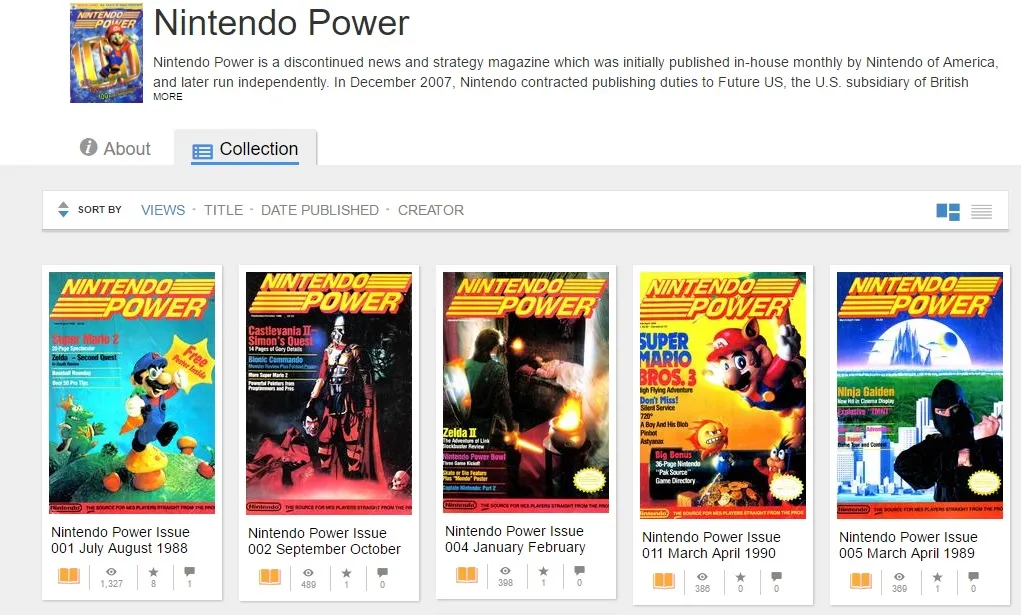The image appears to be a screen capture from a digital archive interface specifically showcasing the iconic Nintendo Power magazine collection. On the left side of the image, there is a graphic featuring Super Mario along with the title "Nintendo Power," referencing the beloved yet now-discontinued monthly news and strategy magazine initially published in-house by Nintendo of America. Later, the publication was handled independently. Below the graphic, text elaborates on the publication's history, noting that in December 2007, Nintendo contracted the publishing duties to Future US, the U.S. subsidiary of a British company.

The interface displays two tabs at the top: "About" and "Collection," with the "Collection" tab highlighted. Below, a taskbar allows users to sort the collection by views, title, date published, or creator, with up and down arrows for easy navigation. The main content area showcases five different cover images of Nintendo Power magazine issues. Two of these covers feature Mario prominently, while the remaining three highlight different game characters.

Each magazine cover also includes the issue number and publication date:
1. The first cover on the far left is labeled "Nintendo Power Issue 1, July/August 1988."
2. The second is "September/October 1988."
3. The third is "January/February 1989."
4. The fourth is "March/April 1990."
5. The fifth cover is "March/April 1989."

This detailed and organized display offers a nostalgic and informative look into the history and legacy of Nintendo Power magazine.